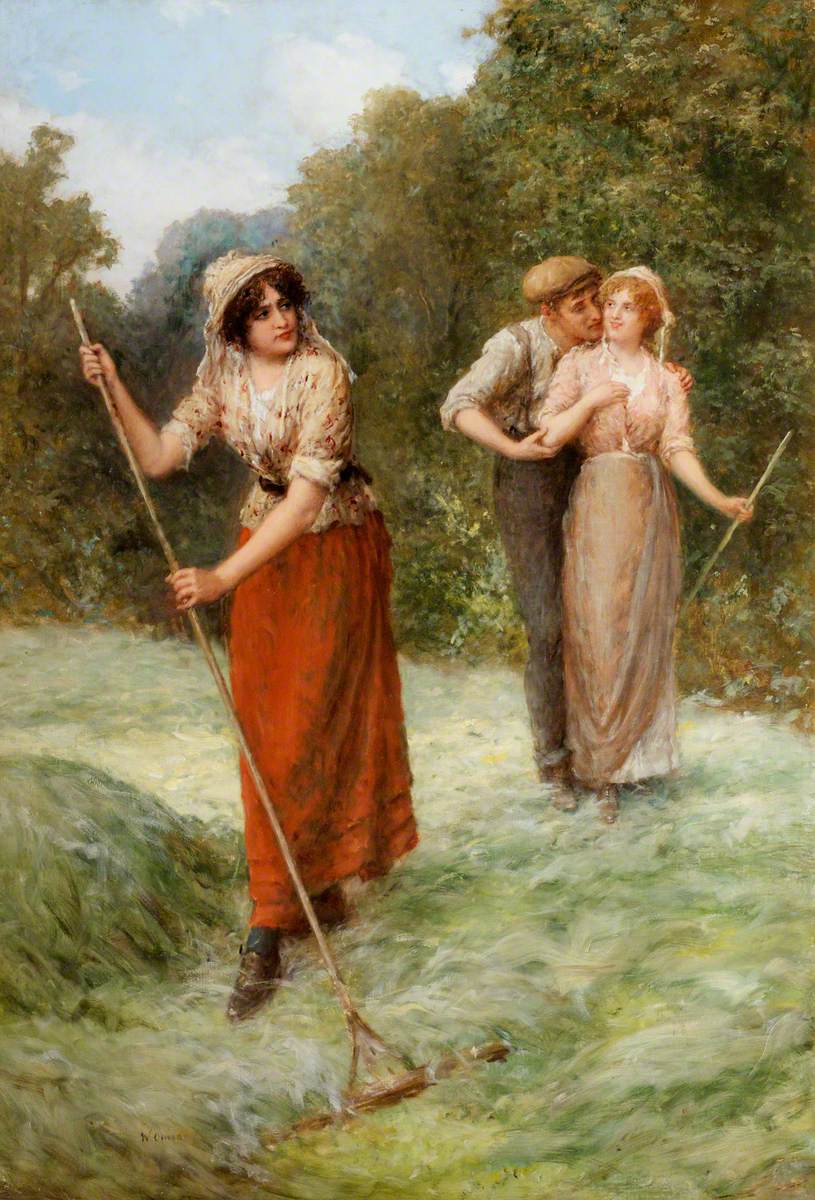In this richly detailed watercolor painting, a woman stands prominently in the foreground, raking wispy grass towards her with a long-handled rake. She wears a burgundy maxi skirt, brown boots, and a belted yellowish top adorned with a red floral design, the sleeves rolled up to her elbows. Her curly brown hair peeks out from under an old-fashioned matching bonnet. She gazes back over her shoulder with a look of disdain.

To the right, in the mid-ground, a man in brown overalls and a newsie cap, paired with a white shirt and suspenders, leans in to whisper into another woman's ear. He grips her left shoulder and right elbow, and her face lights up with a smile. This woman, with strawberry blonde hair and a sheer brown dress revealing a white slip, also holds a rake in her left hand but appears more focused on the man’s flirtations. The overall scene seems to evoke a sense of jealousy or infidelity amidst the serene setting of a grassy field bordered by a tree line beneath a pale blue sky.